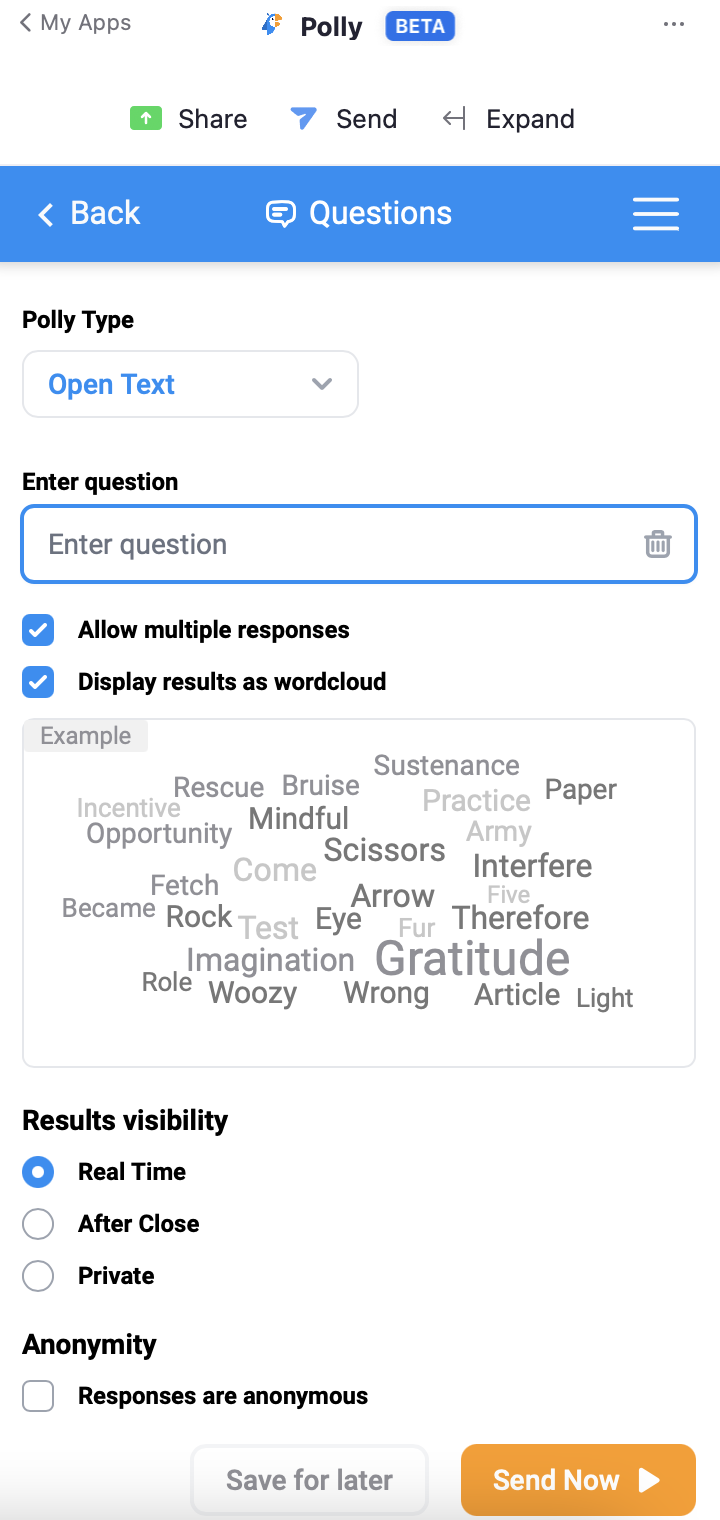The image depicts an interface layout with a blue header section at the top. On the left-hand side of this header, there is a button labeled "Back Questions," while adjacent to it are three horizontal lines stacked vertically, likely indicating a menu icon. Above the header, the word "Poly" is prominently displayed, followed by a smaller blue box labeled "Beta." Below this header, the interface contains buttons labeled "Share," "Send," and "Expand."

Underneath this area, another label "PolyType" is displayed, featuring a drop-down box with the option "Open Text." Further down, there are fields titled "Enter Question" with another drop-down box beneath it also labeled "Enter Question." Below these elements, bold black text reads "Allow multiple responses," with checkboxes next to it and "Display results as word cloud."

At the bottom of the interface, there is a large, rectangular, white background box labeled "Examples." Within this box, various words are scattered, including "rescue," "bruise," "sustenance," "paper," "incentive," "opportunity," "mindful," "interfere," "rock," "I," "therefore," and "gratitude."

This detailed caption provides a comprehensive description of each element visible in the image.